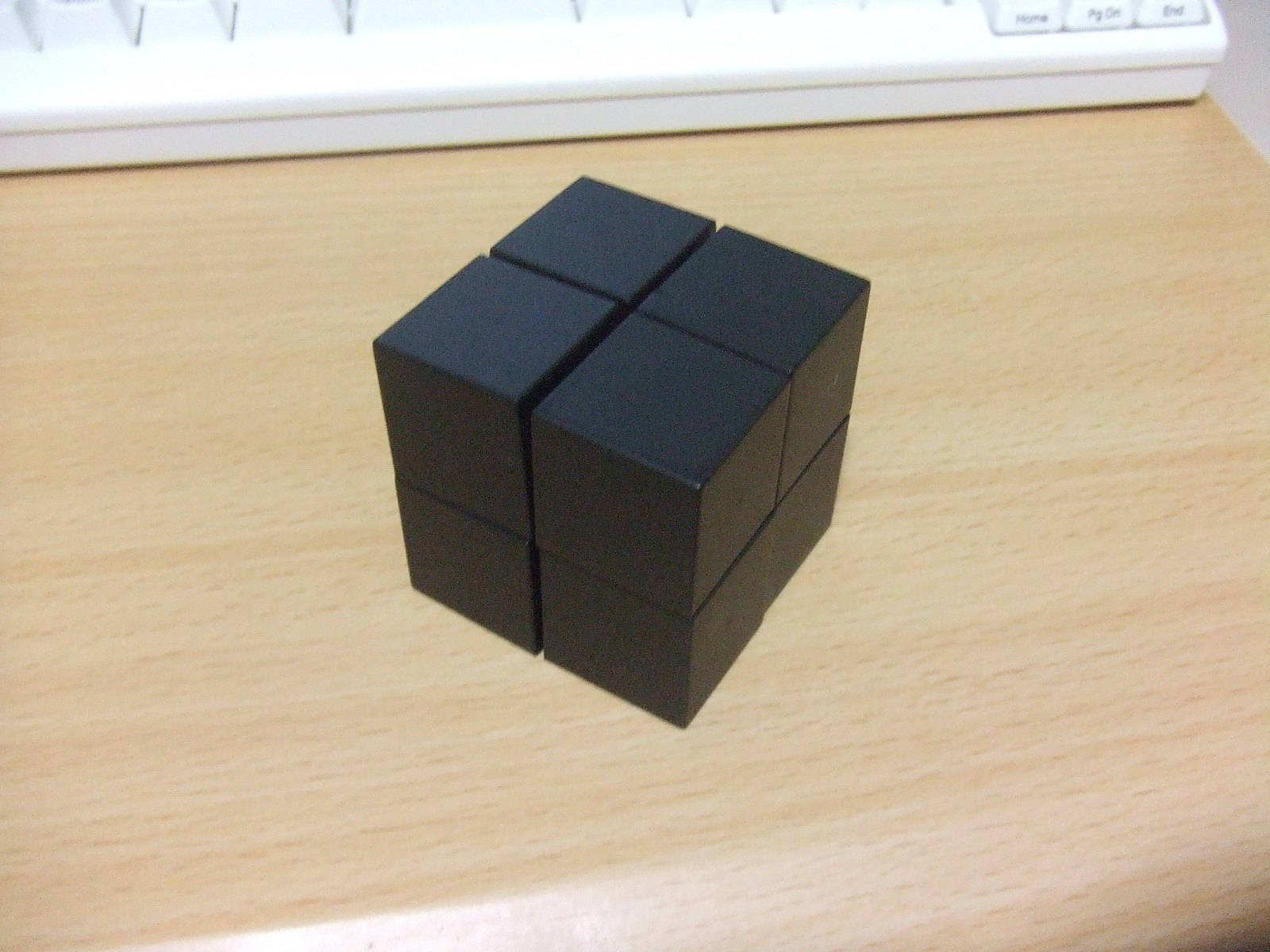The photograph is a close-up of a segmented, jet black cube situated on a light, yellowish-tan wooden table. The cube, which resembles a Rubik's Cube, is composed of smaller cubes with visible gaps indicating separation both vertically and horizontally, forming a grid pattern of four cubes on the top and four on the bottom. The table surface reflects light, hinting at a light source above. In the background, partially obscured yet visible, lies a white keyboard, showcasing keycaps with black text. Specific keys such as "HOME," "PG ON" (likely "PAGE DOWN"), and "END" are discernible. Additionally, the top right corner features a faint gray element, possibly a piece of paper or mouse pad. The overall composition centers the black cube, with the keyboard providing a contextual backdrop.